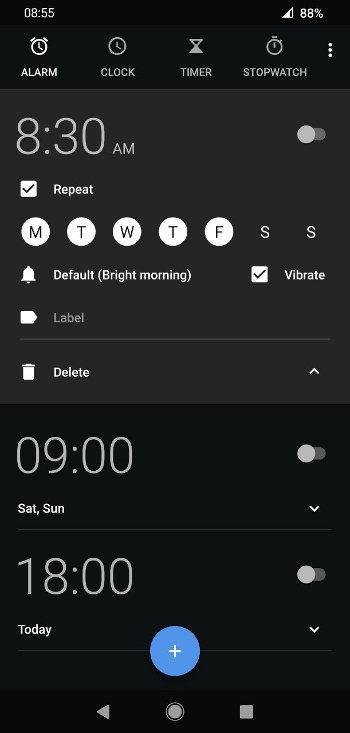In this detailed screenshot of an Android device, indicative of the night theme with predominantly black backgrounds and white or gray text, we can observe several elements. The status bar at the top left displays the time as 8:55, while the top right shows the battery level at 88% alongside the Wi-Fi signal indicator.

Just below, the interface highlights the "Alarm" section within the clock application, which is selected among other tabs like "Clock," "Timer," and "Stopwatch," as well as a menu option represented by three dots for more features. In the "Alarm" section, an alarm is set for 8:30 a.m., scheduled to repeat on weekdays, specifically Monday through Friday, as indicated by the highlighted days. The alarm is set with the default "Bright Morning" sound and has the vibration option enabled. Additionally, there is an option to delete this alarm.

Further down, two additional timers are listed at 9:00 and 18:00. A button with a white plus sign is present, likely for creating new timers. The screenshot also includes the navigation bar at the bottom with the Android standard buttons: the back button, the home button, and the square button for recent apps. The overall dark color scheme suggests the device is in night mode, providing a sleek and subtle visual experience.